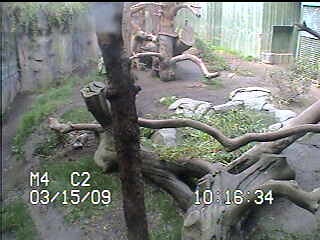The photograph captures what appears to be the aftermath of a storm in a muddy yard, with partial downed trees standing upright but stripped of their limbs as if cut by a saw. The image, timestamped 03-15-09 10:16:34 from a CCTV or security camera, shows two large pieces of what looks like driftwood lying on a dirt surface. Surrounding the dirt are patches of grass ringed with light gray stones. To the left, a tree trunk lies in the foreground, while more green grass and dirt appear to its left. In the distance, on the upper right, stands a wooden structure made of untreated, grayish wood that provides an enclosure with an opening for animals. The upper left corner reveals a fence adorned with fake vegetation. Additionally, the image features on-screen text in white font: "10:16:34" in the lower right corner and "M4C2" along with the date "03-15-09" in the lower left.